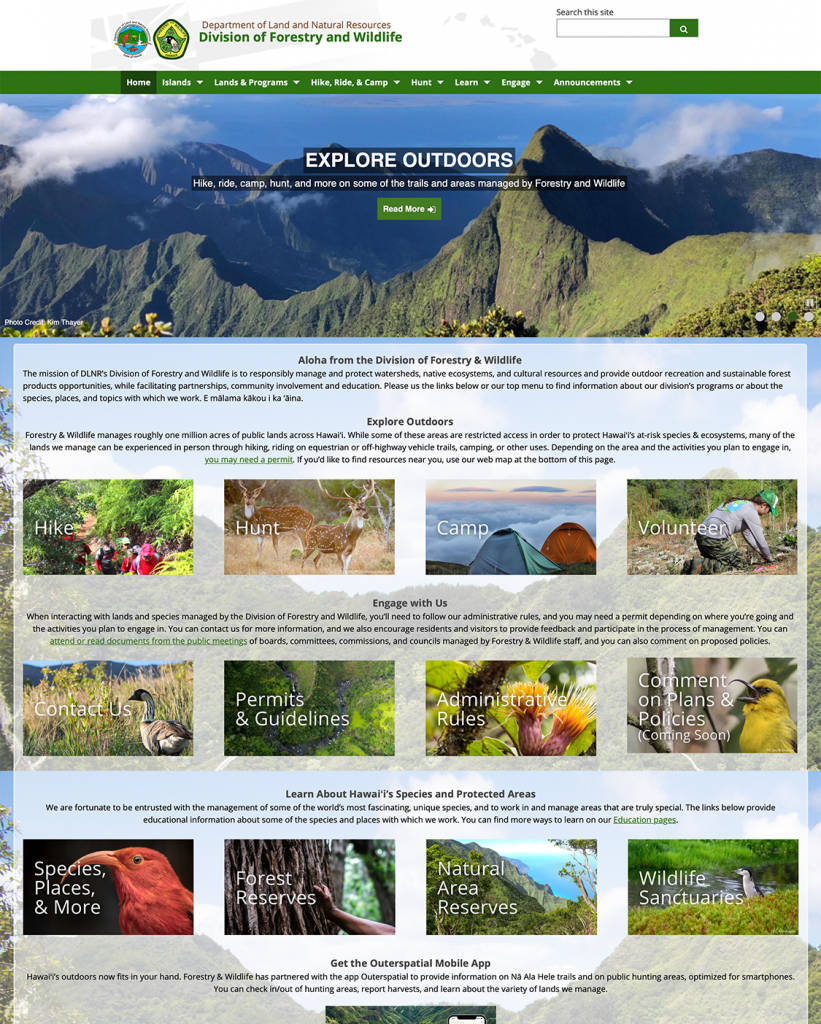This detailed screenshot captures a nature-oriented website, focusing on outdoor activities and featuring various decorative elements. At the top, the header displays two colorful badges—one blue with elements of green and red, and the other green and yellow, potentially hexagonal in shape. Adjacent to the badges is maroon text stating "Department of Land and Natural Resources," followed by bold, green lettering that reads "Division of Forestry and Wildlife." In the upper right is a search bar, characterized by a white background, black outline, and a green button housing a white search icon, complemented by the text "search the site" above it. The background of the header is predominantly white, accentuated with light gray silhouettes that resemble either the Earth or a country.

Below the header is a green navigation bar that spans the website's width, featuring small, legible links: Home, Islands (with a drop-down menu), Lands and Progress (with a drop-down menu), Hike, Ride, and another option (with a drop-down menu), Learn, Engage, and an option beginning with 'A'. 

The Hero section comprises a striking mountain range image, with earthy tones of brown and black and lush greens at the bottom, under a clear blue sky. Centralized in this section is bold, white text reading "Explore Outdoors," enclosed by a slightly larger black overlay, providing contrast. Beneath this, a subheading in small, white text follows the same overlay design, accompanied by a green button labeled "Find More."

The main body of the site kicks off with a welcoming message: "Aloha from the Divisions of Forestry and Wildlife," followed by an unreadable three-line paragraph. Next, another header "Explore Outdoors" is followed by another three-line paragraph, leading to a row of four images with overlaid text: "hike," "hunt" (depicting deer), "camp" (illustrating tents in a cloudy area), and "volunteer" (showing a person engaged in a nature-related task). This pattern repeats with sections of subheadings, small text, and sets of four images with white text overlays.

The image ends with a final section featuring another subheading and just one cut-off image beneath it. This entire section sits on a semi-transparent white overlay, offering a glimpse of the underlying picture, contributing to the visually rich and busy appearance of the website decorated with numerous nature photos.